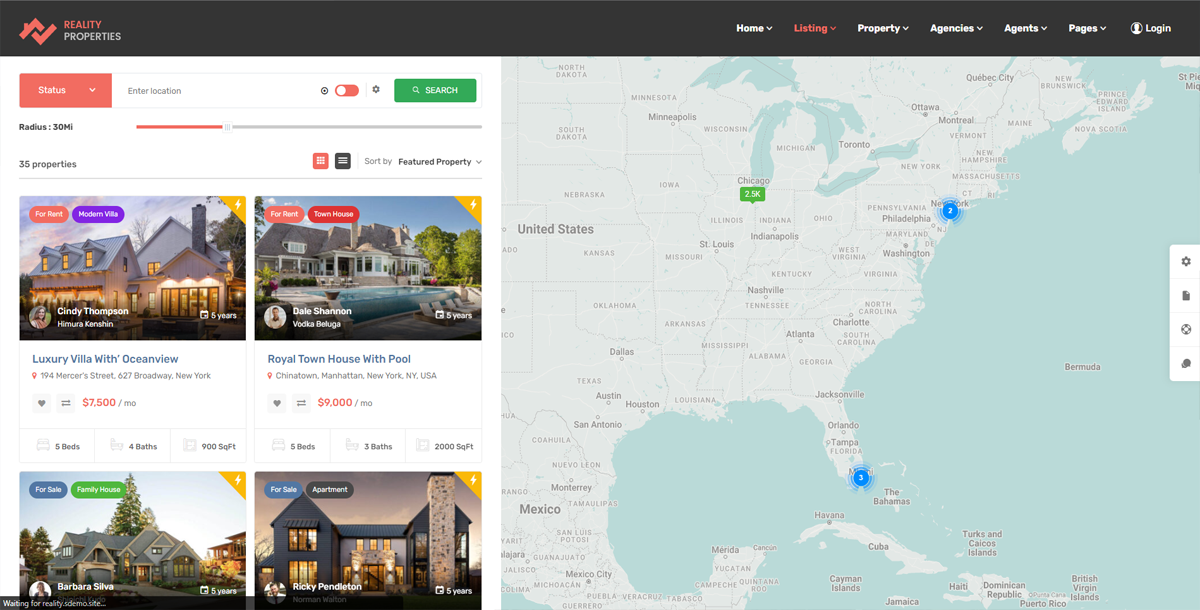Here is a detailed and cleaned-up caption based on your description:

---

This color screenshot showcases the homepage of the "Reality Properties" website. At the top, a black banner prominently displays the site name "Reality Properties," followed by navigation links such as Home, Listing, Property, Agencies, Agents, Pages, and Login on the right side. 

On the left, there's a search interface with options including Status, Enter Location, Search, Radius (30 miles), 35 Properties, and Sort by Featured Property. 

Below are several property listings with accompanying photographs:
1. A large, two-story white house marked "For Rent." The description reads: "Modern Villa by Cindy Thompson and Himura Kenshin, 5 years. Luxury Villa with Ocean View located at 194 Mercer Street, 627 Broadway, New York. Priced at $7,500 per month, offering 5 beds, 4 baths, and covering 900 square feet."
2. An image of a house with an outdoor pool labeled "For Rent." The description states: "Townhouse by Dale Shannon and Vodka Beluga, 5 years. Royal Townhouse with Pool situated in Chinatown, Manhattan, New York, NY, USA. Priced at $9,000 per month, featuring 5 beds, 3 baths, and encompassing 2,000 square feet."
3. A two-story house with trees in the background tagged "For Sale." The visible details read: "Family House by Barbara Silva, 5 years." The rest is cut off at the bottom.
4. A two-story dark gray house with a stone chimney listed "For Sale." The available description includes: "Apartment by Ricky Pendleton, 5 years." The remainder is cut off at the bottom of the image.

To the right, there is a map of the United States, which seems intended for property location purposes.

---

This detailed caption provides a clear and structured summary of the screenshot's content, ensuring the reader understands each element's context.